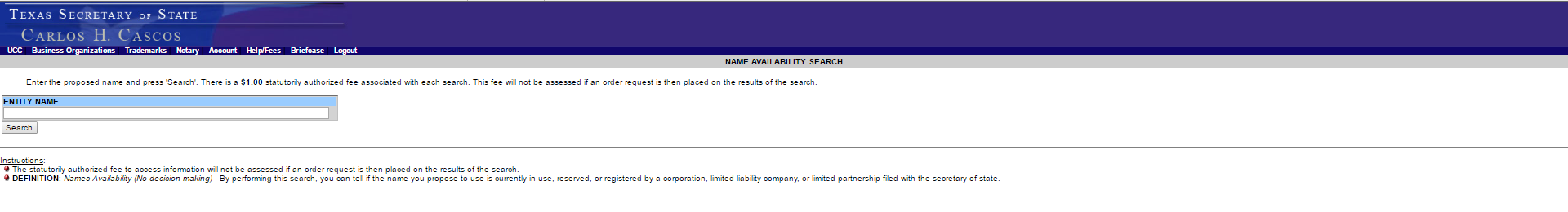The image depicts the magnified top section of the Texas Secretary of State website, overseen by Carlos H. Cascos. The screenshot, enlarged to 250% for clarity, features a navigational bar that includes links to UCC, business organization, trademarks, notary, account, help, briefcase, and logout functions. A highlighted instruction reads, "Enter the proposed name and press search," with a notification that a statutory fee is associated with each search, although this fee will be waived if an order request is made based on the search result.

Centered above this instruction is a light purple stripe with the text "Name Availability Search." Below this, a blue-highlighted section instructs users to input the "entity name" in the designated search field and then press "search." Additional instructions follow, though the text becomes increasingly small and less readable.

The overall design facilitates name searches within the Secretary of State's business-related databases, ensuring clarity and ease of use for individuals seeking information.